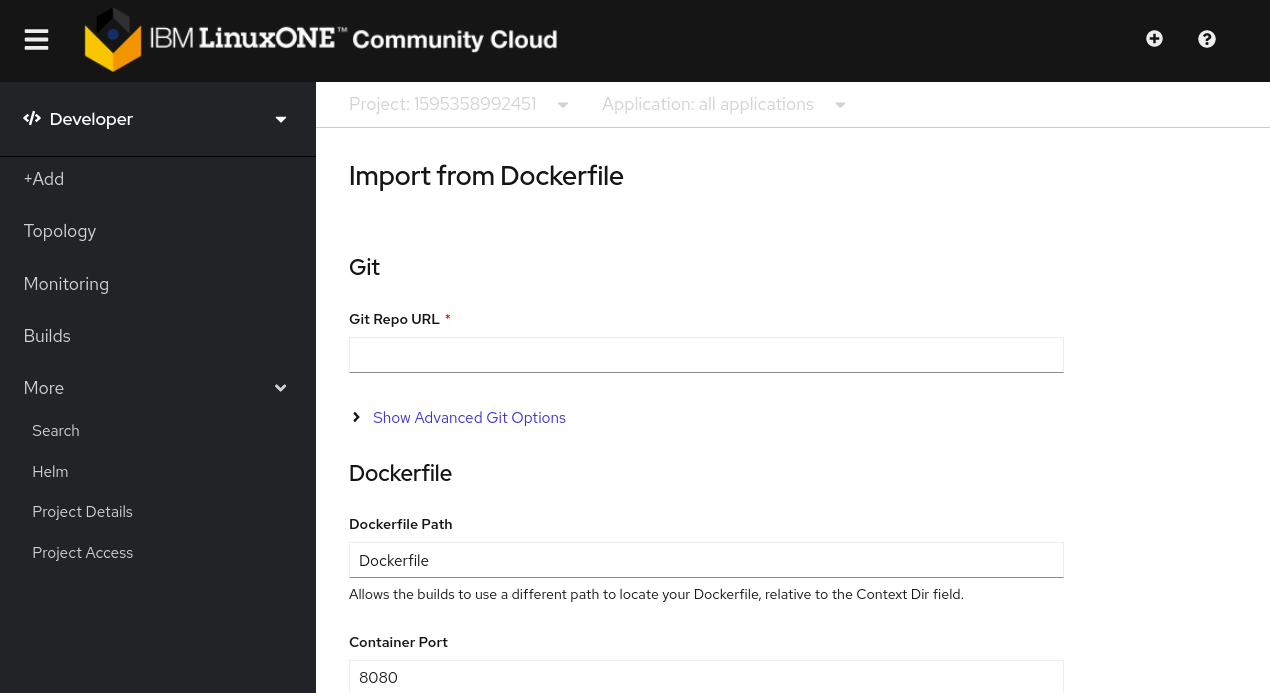The image showcases the IBM LinuxONE Community Cloud interface. On the left sidebar, a vertical stack of menu options is visible, starting with "Developer," followed by "Add," "Topology," "Monitoring," "Builds," and "More." To the right, there is a search bar and options such as "Product Details" and "Project Access."

Central to the image, a drop-down menu labeled "project-1-5-9-5-3-5-8-9-9-2-4-5-1" is present, alongside another drop-down menu titled "All Applications." Below these, there is an option to "Import from Dockerfile." Further down, the interface prompts for a "Git Repo URL" with a red asterisk indicating a required field, followed by a divider line.

Additional sections include "Show Advanced Git Options," "Dockerfile," and "Dockerfile Path." The Dockerfile path description indicates it allows builds to use a different path to locate the Dockerfile relative to the context directory field. To the right, specific container details such as "Container port 8080" are mentioned, signifying a website or application for the community cloud project.

The overall background of the interface is white, providing a clean and structured layout for project management and development within the IBM LinuxONE Community Cloud environment.